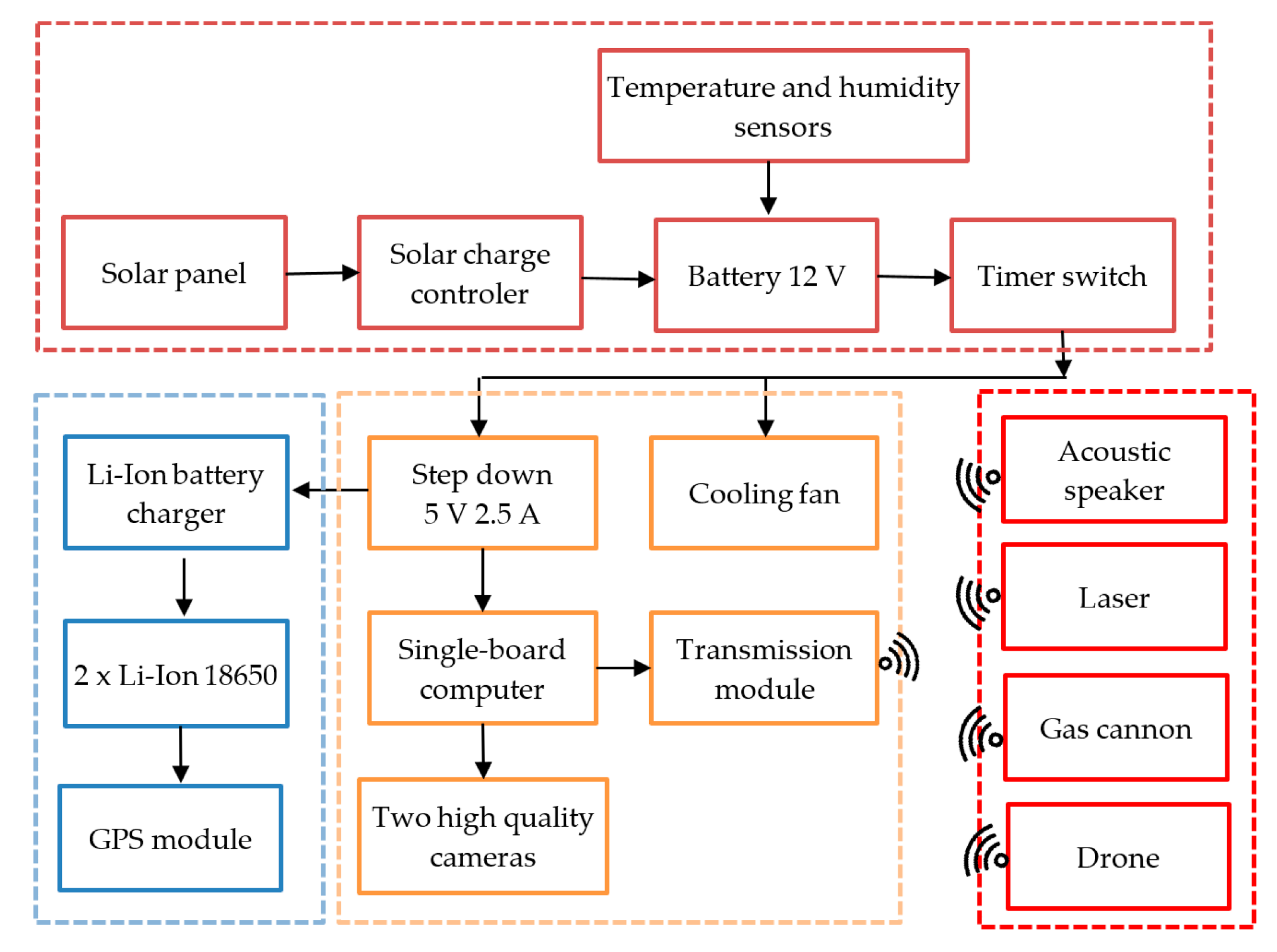The image depicts a detailed flowchart set against a white background. The chart consists of one horizontal rectangle at the top, followed by three vertical rectangles beneath it, each containing smaller labeled rectangles with black text. Directed by black arrows indicating the sequence, the flowchart begins with "temperature and humidity sensors" and proceeds to "solar panel," "solar charge controller," "battery 12V," and "timer switch." From the timer switch, the chart branches out to multiple components: a "step-down 5V 2.5A" module leading to a "single board computer," which in turn connects to "two high-quality cameras," a "cooling fan," and a "transmission module." Another branch directs to an "Li-ion battery charger," which feeds into "2x Li-ion 18650" cells and subsequently a "GPS module." The rightmost section identifies additional components such as an "acoustic speaker," "laser," "gas cannon," and "drone," illustrating a comprehensive and interconnected system.